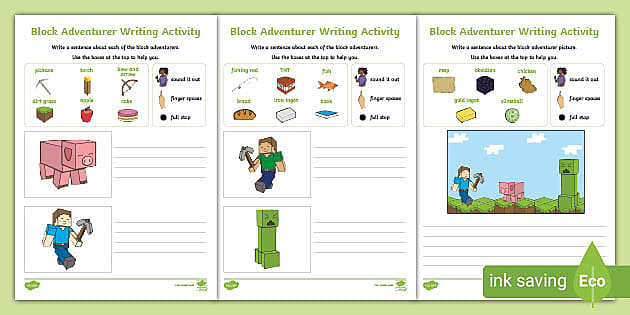This image is a detailed, color-illustrated, landscape-oriented graphic showing three side-by-side workbook pages from an elementary textbook, each bordered by a light green color. The heading at the top of each page reads "Block Adventurer Writing Activity" in green letters. Below the headings are various sections featuring colorful illustrations and diagrams related to the Minecraft game, such as tools and objects like an ice pick, apple, fish, white cube, blue cube, bread, and more.

Each page is structured similarly with images on the left and blank lines or columns on the right for writing activities. On the left page, colorful icons like a pickaxe, bow and arrow, and a block pig are displayed, accompanied by writing lines. The center page features a man carrying an axe, dressed in green, and below him, a block robot, both with designated writing lines. The right page includes items like a button, cube, calcium block, butter block, and another depiction of the block robot and person in a field.

The images and icons are interspersed with directions for the writing activities. Additionally, a green horizontal band with white text reading "Ink Saving Echo," alongside a green leaf icon, is present in the bottom right corner. The style combines elements of color illustration, graphic design, and typography.